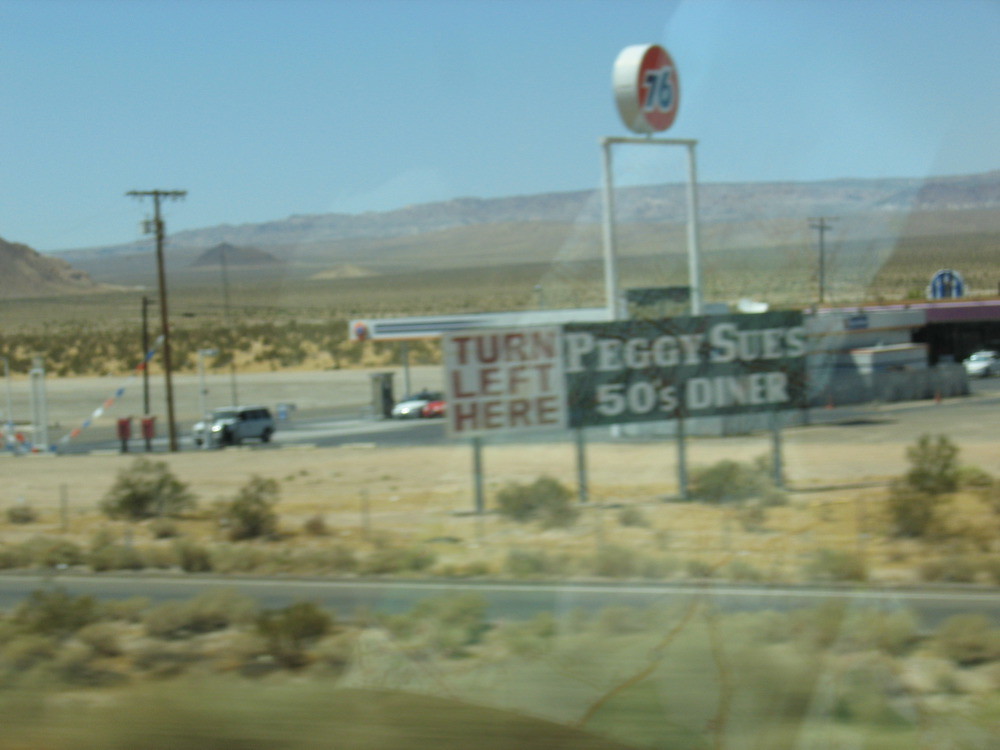This photograph, taken from inside a vehicle through a window, exhibits a faint reflection of a white sleeve across the image. The scene captures a desert or really dry climate characterized by sandy soil and sparse, small shrubs. The foreground features a road running left to right, leading to a 76 gas station and Peggy Sue's 50s Diner. The station is adorned with a prominent, round 76 sign supported by two vertical poles, and a larger rectangular billboard. This billboard, mounted on four vertical poles, is split into a white section reading "Turn Left Here" and a black section advertising "Peggy Sue's 50s Diner." The background reveals a vast, barren landscape with few vehicles, public telephones, and electrical poles. Tall, brown mountain ranges and a bright blue sky with minimal vegetation enhance the backdrop, capturing the essence of this arid locale.